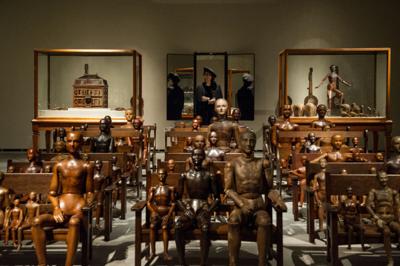The photograph captures an intricate art installation in a museum room. The centerpiece of the exhibit features numerous wooden carved figures, ranging from adults to children, arranged in three rows of benches that resemble either an old church or a historical schoolroom. The wooden figures vary in shades, from light to dark, and are meticulously detailed, displaying ball and socket joints at the knees and elbows, with carved faces and anatomical features, all seated in natural, unclothed states. 

In the background, the room is dim, except for two spotlights illuminating two distinct glass cases. The left case houses a detailed sculpture resembling a Dutch-style building with a brown roof. In the right case, a wooden figure is displayed, depicted in a dynamic pose with one knee raised. Between these cases, a large triptych painting or mirror is mounted on the wall, showing figures oriented in differing directions. Standing near the back wall is a woman dressed in a black beret and black jacket, observing the exhibit. The room's dark ambiance is enhanced by the gold metal borders framing the glass cases, adding a touch of elegance to the scene.